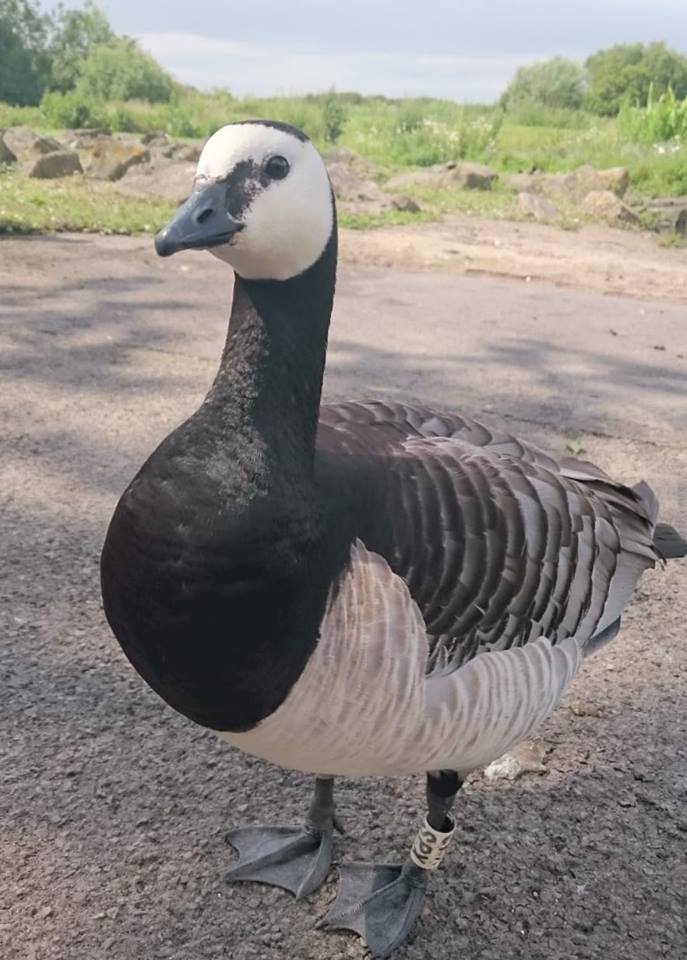This highly detailed, realistic photograph is vertically oriented, recorded during the day with good lighting under a light blue sky scattered with white clouds. The vibrant background features lush green grass, several trees, and some rocks, giving a natural landscape setting. The foreground shifts to a cement or tightly packed dirt lot, where a striking waterfowl, resembling a goose, stands poised.

The bird is predominantly black and white, with its striking white face and stomach contrasting against the black that adorns its neck, back, and wings. Its webbed feet are visibly black, and it bears a small cylindrical tag with numbers on its left leg. The bird also has a black beak and black eyes, and it's gazing towards the left side of the image. The feathers are lined and sleek, close against its body, blending various shades of black and gray, especially around its tail area. The bird stands elegantly, creating a captivating focal point against the mixed terrain of dirt and rocks enveloped by the greenery.